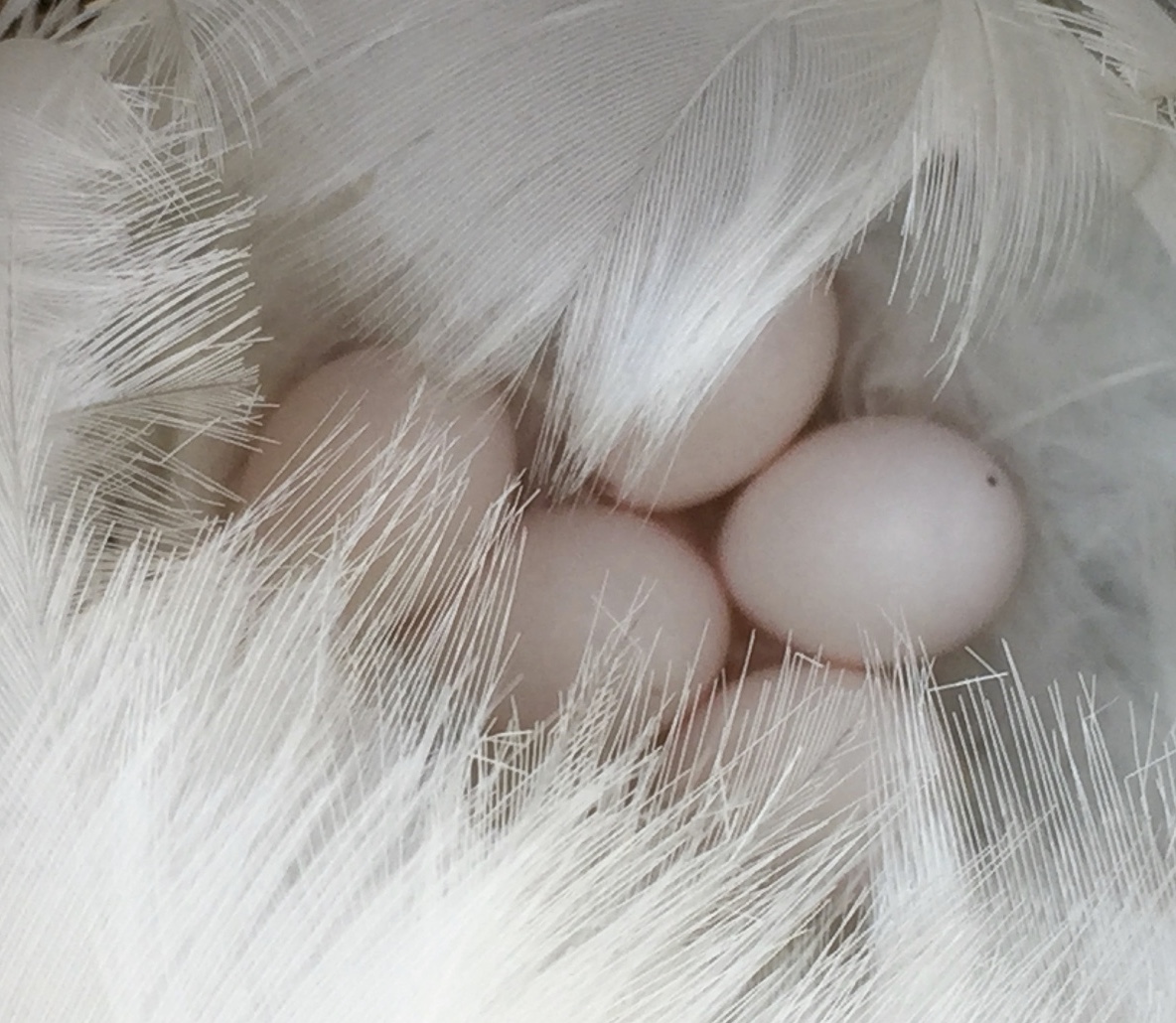The image showcases five very light pink eggs that are meticulously nestled within a bed of pristine white feathers. The feathers envelop the eggs from the top, sides, and bottom, leaving only the rightmost egg partially uncovered, distinct with a tiny black spot on its surface. The white feathers create a delicate, almost pillowy cradle for the eggs, suggesting a possible decorative or thematic arrangement, perhaps for an Easter display. There's a gentle interplay between the stark whiteness of the feathers and the softer white of the underlying material, adding to the overall serene and delicate ambiance. The exact nature of the eggs—whether real or artificial—and the origin of the feathers remain ambiguous, adding an element of mystery to this elegantly arranged scene.